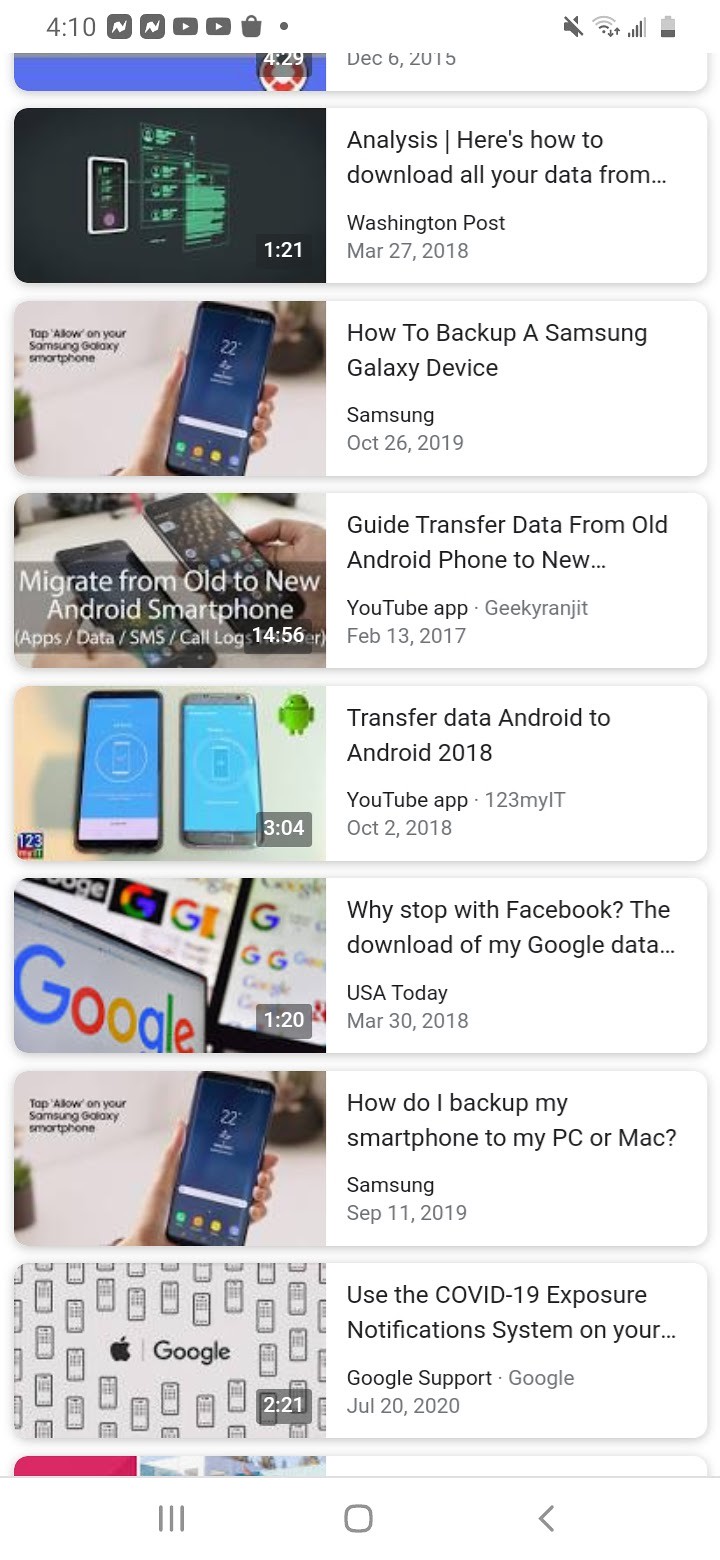The image appears to depict a search engine interface on a computer or smartphone. At the top, there is a search bar with the keyword "analysis" entered. Above this, a small indicator displays the number "410." The interface is populated with several small icons and features a blue stripe containing a circular emblem with red and white colors.

Below this, the image shows a series of search results in white text boxes bordered by light gray. The first entry indicates an article titled "Here's how to download all your data from" by The Washington Post. The subsequent entries, also in blue text, include guides such as "How to back up a Samsung Galaxy device," "Guide: Transfer data from old Android phone to new," "Transfer data Android to Android 2018," "Why stop with Facebook to download my Google data" from USA Today, "How do I back up my smartphone to my PC or Mac," and an instruction from Google Support on "Use the COVID-19 exposure notification system." A small black image or icon is visible alongside the text, along with a green light or indicator next to the word "analysis."